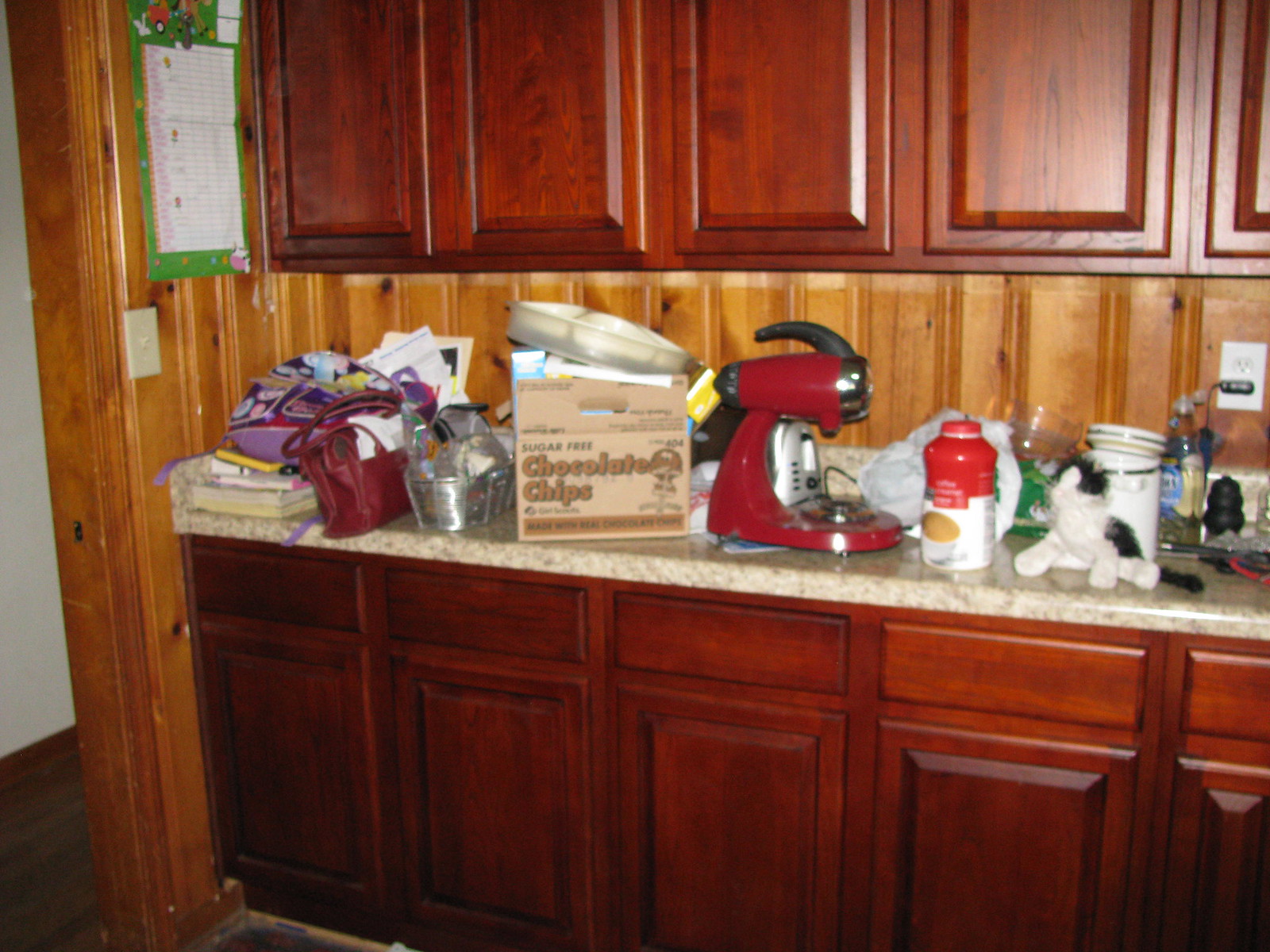In the image, a kitchen is prominently featured with dark brown cabinets and a striking white marbled countertop. Medium-colored wood paneling forms the backdrop, adding a warm and inviting atmosphere. The countertop is cluttered with various items, drawing the eye toward an old-fashioned, red stand mixer at the center. This classic mixer, designed to hold a bowl that turns itself during operation, evokes a sense of nostalgia.

To the left of the mixer, there's a notable large cardboard box labeled "chocolate chips." Adjacent to this box are a couple of unsorted bags and a stack of paperback books, which appear to be cookbooks, although their titles are not visible. To the right of the mixer stands a bottle that resembles V8 juice, hinting at a potential ingredient choice for whatever is being prepared.

Adding a whimsical touch, a stuffed cat toy with a white body and paws and a black head, back, and tail is propped up beside the bottle. Further in the background, a ceramic canister and a clear plastic water bottle complete the scene, suggesting a kitchen that is both functional and filled with personality.